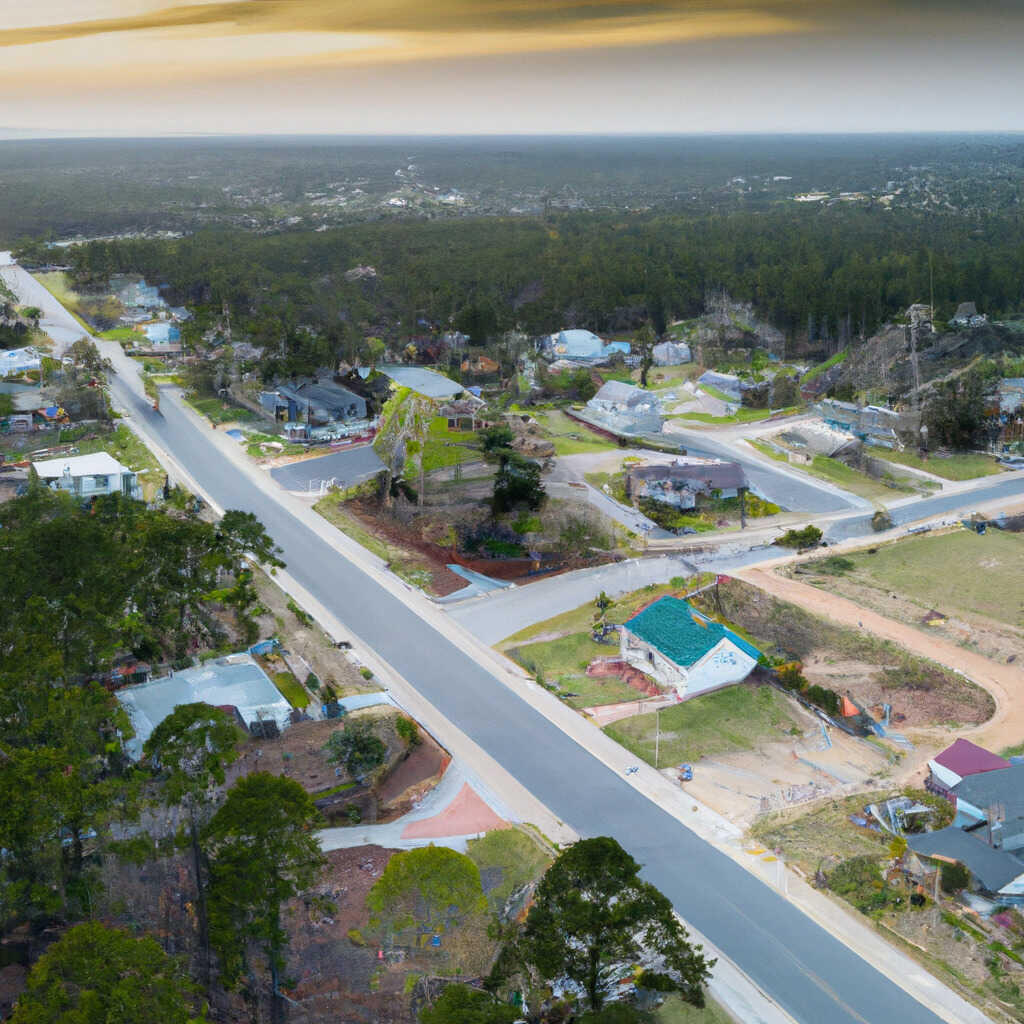This aerial photograph captures a serene residential neighborhood at dusk. The view, taken from high above, showcases an intricate grid of streets branching off the main gray road that bisects the scene. Houses of various designs and roof colors—ranging from bright green to blue and gray—line both sides of this primary thoroughfare. The lots vary in size, with some homes nestled amid clusters of trees, offering a mix of green canopies and landscaped yards. One notable house on the right side features a distinctive blue roof. Flanking the residential area, a dense tree line and expansive fields create a natural boundary, further emphasized by the silhouette of distant hills or mountains against the backdrop of a setting sun, casting a warm glow over the tranquil scene. The overcast sky hints at a peaceful evening, enhancing the rural ambiance of this secluded neighborhood.